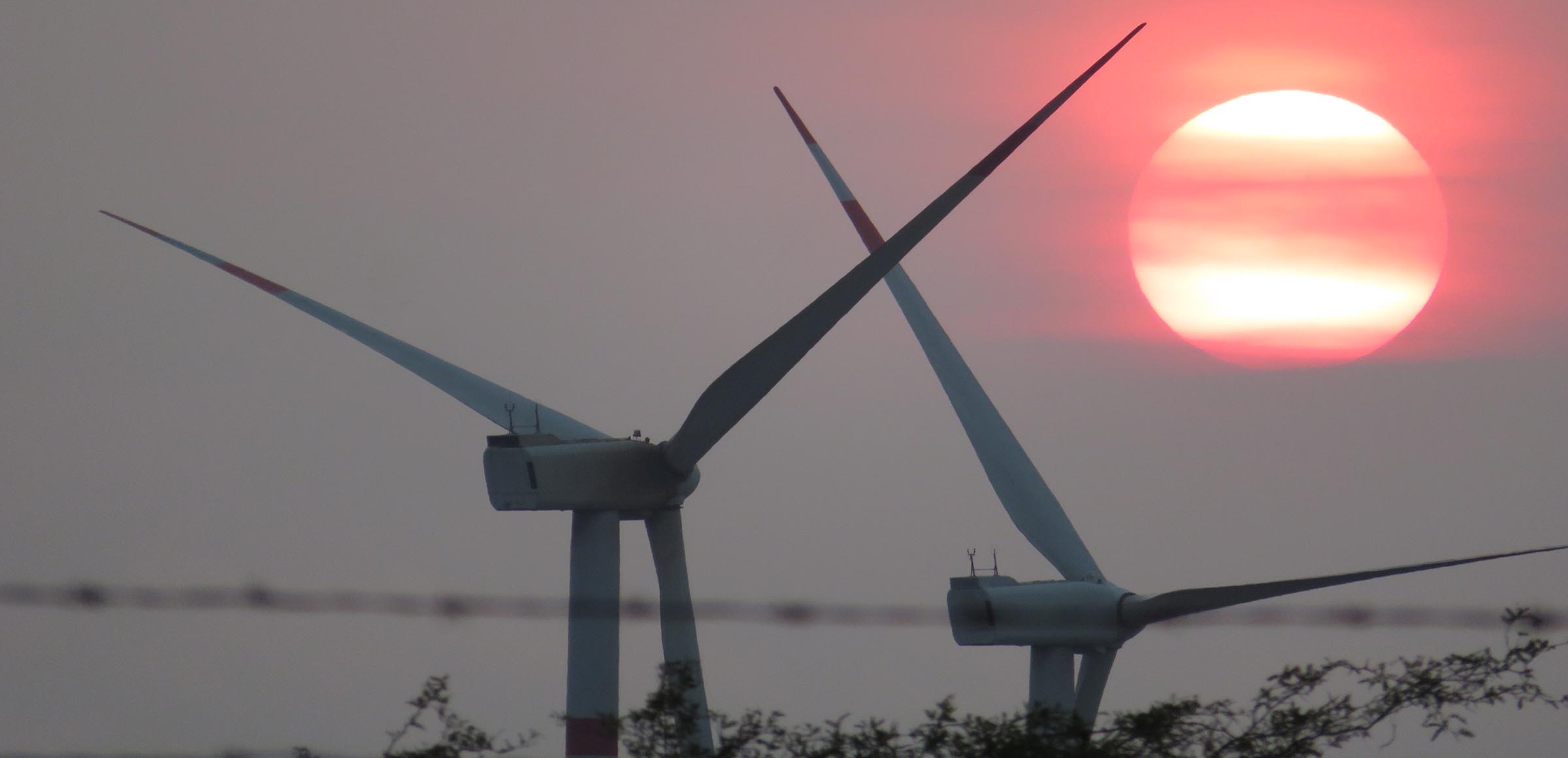Against the gray backdrop of an overcast sky, this photograph captures the top portions of two tall wind turbines from behind. Each turbine sports three long, white blades extending from their crosswise-mounted motors atop towering poles, reminiscent of those seen in Palm Springs, California. In the upper right corner, a large sun, shrouded by orange-tinted, hazy clouds, appears to be setting, casting a light yellow, almost white hue with an orange halo around it. Near the bottom of the image, out-of-focus barbed wire and spiky branches or vines are faintly visible, hinting at the photographer's vantage point behind a barrier. The overall scene is one of serene, industrial presence against a somewhat mystical, dusk-lit landscape.